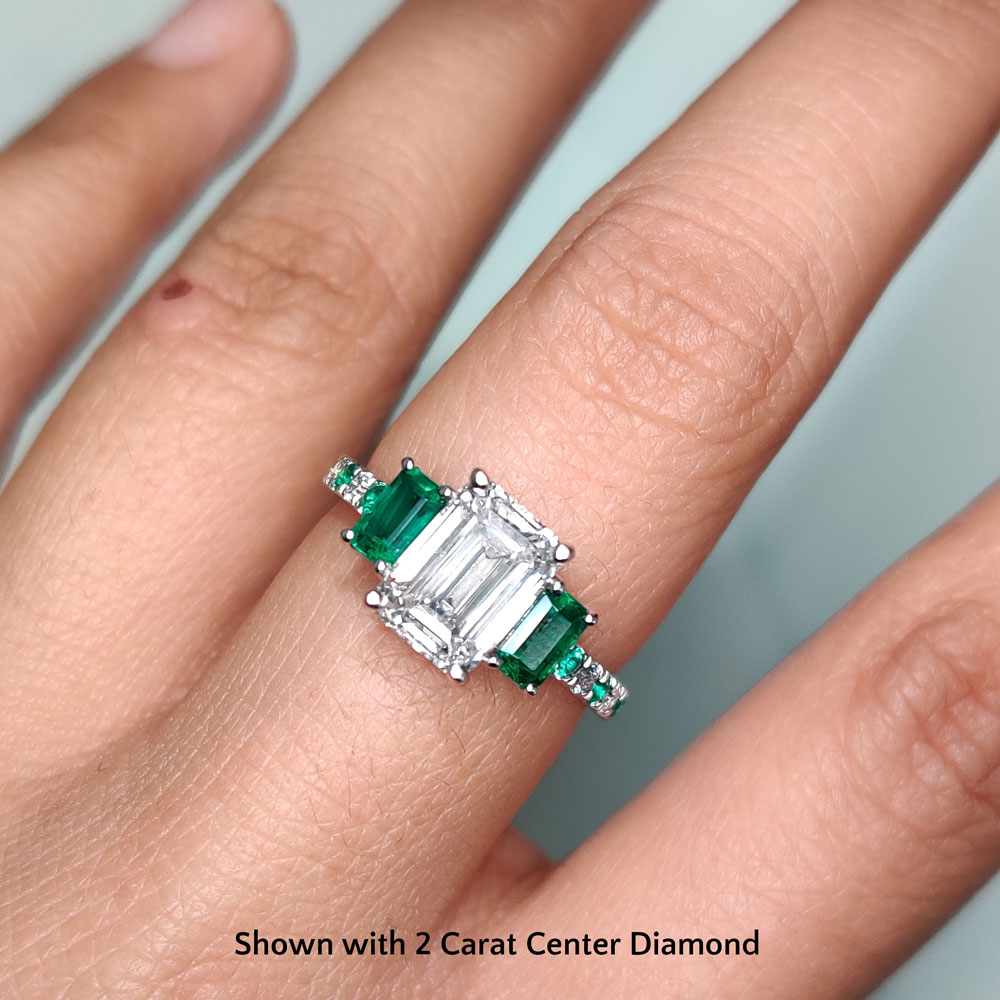This photograph presents a detailed close-up of a white woman's hand, primarily focusing on the four fingers from the index to the little finger against a white background. The centerpiece of the image is an exquisite ring on the middle finger. This stunning piece of jewelry features a large, square-cut, two-carat diamond at its center, elegantly flanked by two substantial emeralds. The band itself is intricately designed, adorned with alternating smaller emeralds and diamonds that cascade towards the bottom of her finger. Visible are the hand's wrinkles, drier skin, a few dings, and cuts. Notably, on the ring finger, there is a small red birthmark on the knuckle. Text at the bottom of the image reads, "shown with two carat center diamond," emphasizing the grandeur of the central gem.